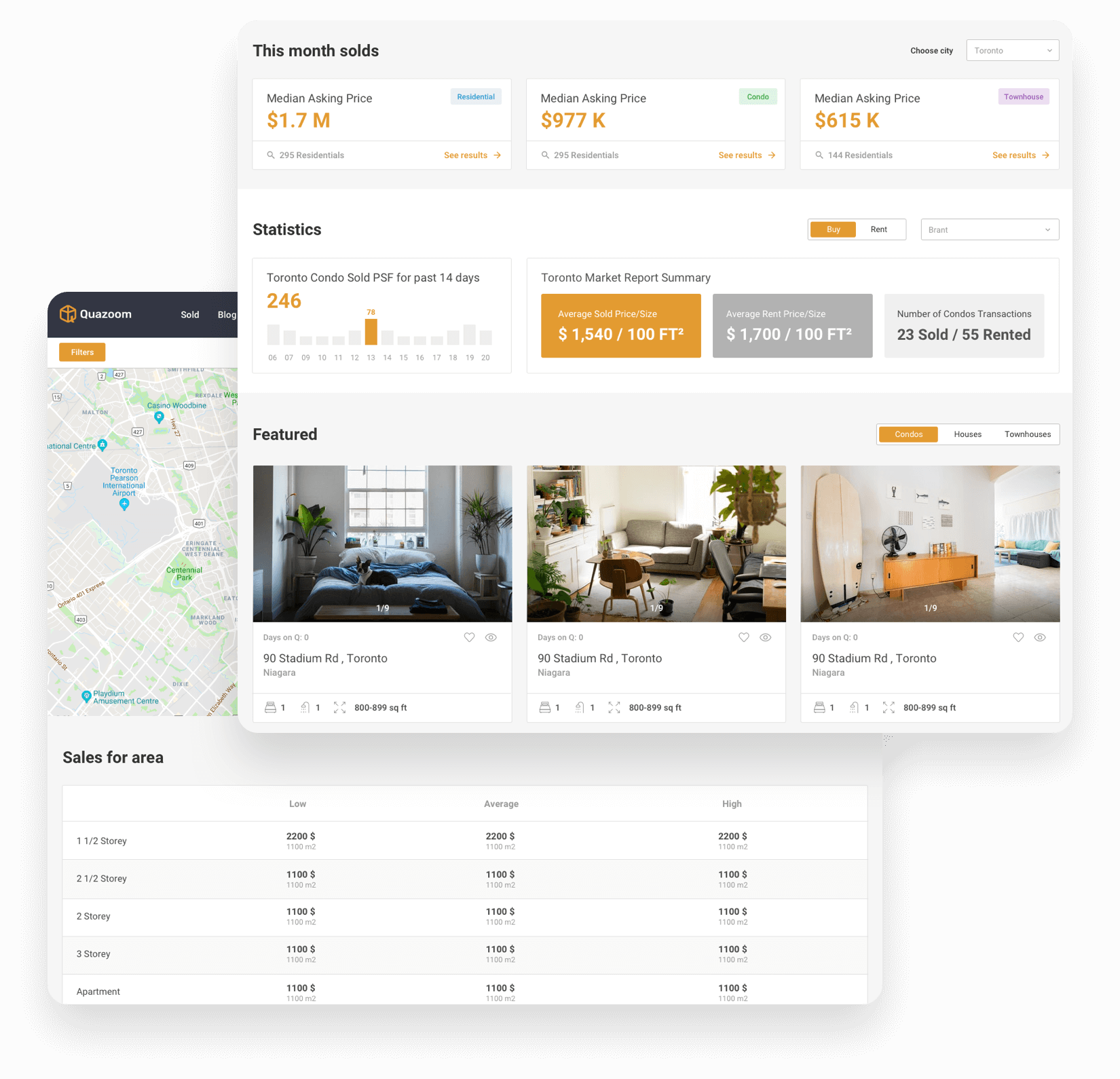The image depicts two overlapping web pages, one positioned at the upper right and labeled "This Month's Solds." This page showcases various real estate statistics, including three distinct median asking prices displayed in white squares: $1.7 million, $977,000, and $615,000, sequentially from left to right. Below these figures is a statistics section highlighting that 246 condos have been sold in Toronto. At the bottom of the page, there are three rectangular blocks, each illustrating different condos in Toronto. Each block includes details such as the condo's address, the number of bedrooms, and the number of bathrooms. The overlapping web page beneath is slightly positioned to the upper left, hinting at additional content not fully visible due to the overlay of the foremost page.